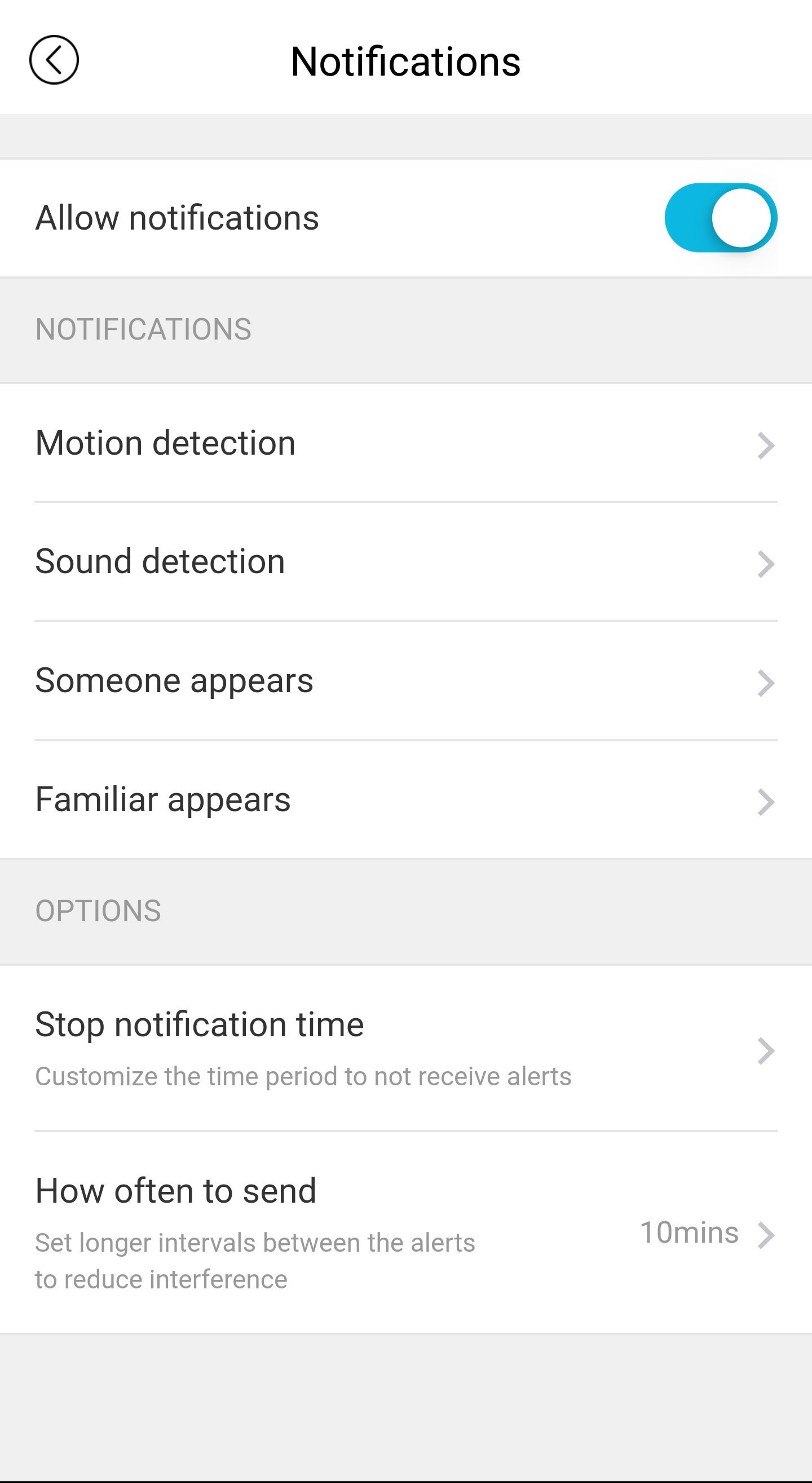Screenshot of the Notifications Settings Page on a Smartphone

The screenshot displays the notifications settings page on a smartphone. At the top of the screen, a header is present with the text "Notifications" centered in black font. To the left of the header, there is a bubble icon with a left-facing arrow.

Below the header is a light gray section followed by a white section with the text "Allow Notifications" accompanied by a toggle switch, which is in the "on" position.

Underneath, another light gray section is labeled "Notifications." This is followed by various options, each with a right-facing arrow to their right. These options include:

- "Motion Detector"
- "Sound Detection"
- "Someone Appears"
- "Familiar Appears"

Each option is separated by light gray sections.

Further down, there is a gray box labeled "Options," with a white box underneath it labeled "Stop Notification Time." This section includes gray text that reads, "Customize the time period to not receive alerts," and a right-facing arrow on the far right.

Below this is an option labeled "How Often to Send," accompanied by gray text stating "Set longer intervals between the alerts to reduce interference." To the right, it reads "10 minutes" followed by a right-facing arrow.

Finally, the page ends with an empty light gray box. The screenshot is a comprehensive view of the various notification settings available on the website's notifications page.